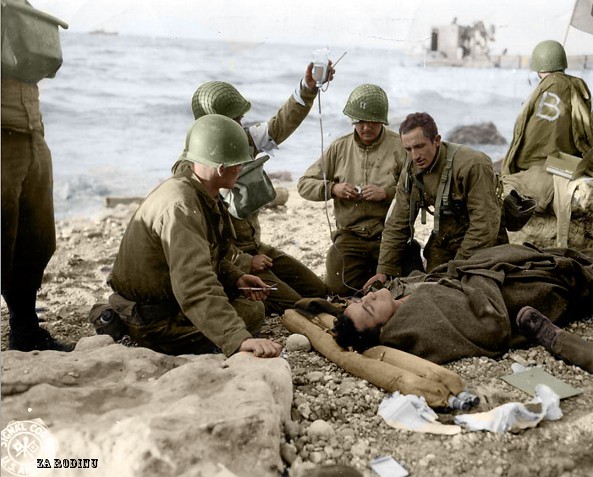In this slightly wide rectangular photograph from what appears to be World War II, a group of six soldiers are gathered around a fallen comrade in a poignant scene set on a gray, rocky terrain. The image, although slightly grayed, is still in color. In the background, there is a light blue sea and, in the distance to the right, a gray battleship or submarine can be seen. The soldiers, all males, are dressed in green uniforms with dark green helmets—except for one concerned soldier leaning over the injured man with his helmet off. The fallen soldier, who has dark hair and light skin, is lying on a dark gray blanket with his head resting on two long, brown pillows or perhaps rolled-up burlap. One soldier in the center is holding an IV bottle that is connected to the injured man's arm, while another is handling a needle, and a third is getting some tape. On the far right, a soldier in a green cape marked with a large letter 'B' is sitting on the rocks, looking into the distance. Another soldier standing to the left has backpack straps visible over his uniform, which also sports a front pack. A man wearing glasses, identified as a lieutenant or captain by the symbol on his helmet, also features prominently. Small lettering at the bottom left of the photo reads "Z-A R-O-D-I-O-U."